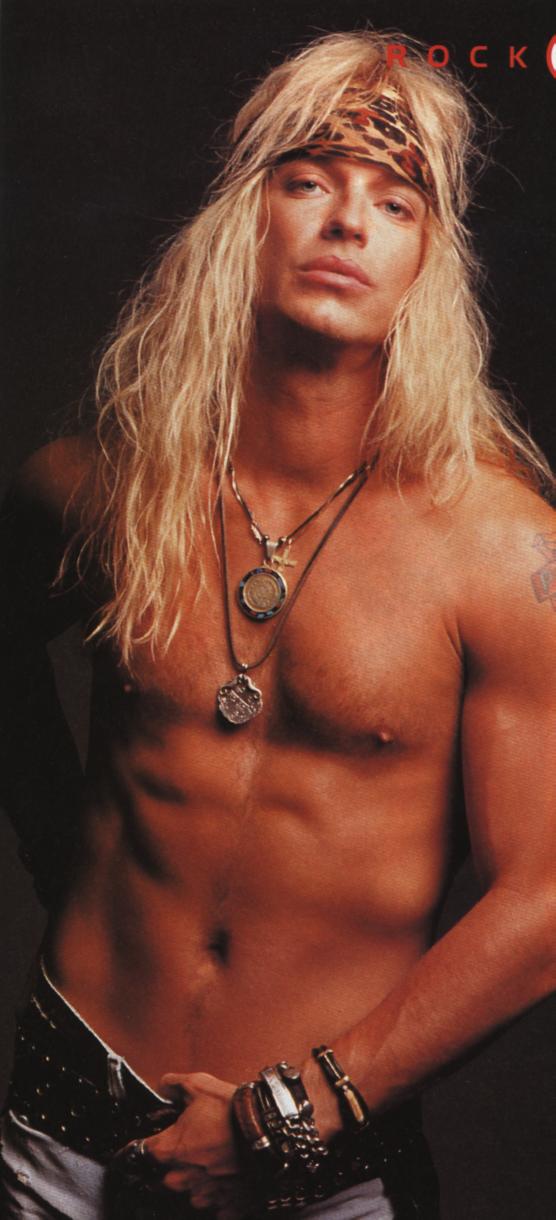In this image, likely depicting either Axl Rose from Guns N' Roses or Brett Michaels from Poison, we see a shirtless rock singer with long, chest-length, stringy blonde hair. The individual sports a tan leopard print headband around their forehead and multiple pieces of jewelry, including two necklaces with pendants, several bracelets on their left wrist, and a ring. Their left shoulder, visible to the viewer, showcases a tattoo. The singer is dressed in light-colored pants with a dark belt, and their left hand appears to be gripping the belt suggestively. The right arm is hidden behind their back. The image is vertical, with the word "ROCK" in red letters at the top right corner.